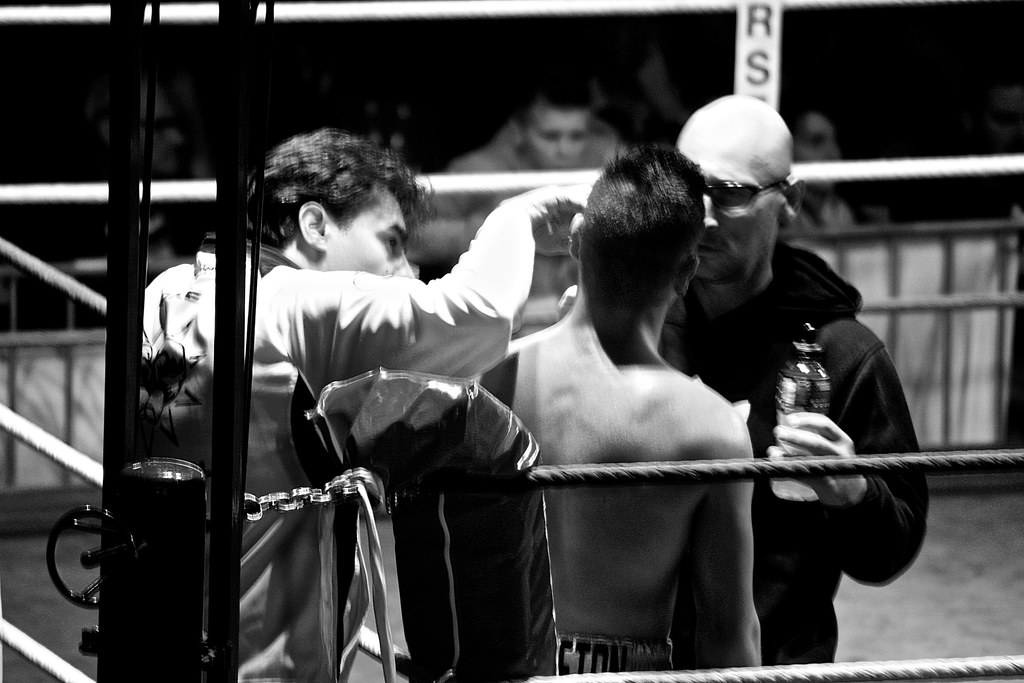In this captivating black and white photograph taken during a boxing match, the scene focuses on a key moment between rounds in an indoor gym. Centered in the near left corner of the ring, the composition prominently features the turnbuckle and two white ropes extending out horizontally across the bottom of the image, held in place with a sturdy chain. 

A boxer, sitting on a stool with his back against the turnbuckle, is the primary focus. Bare-chested and clad in shorts with an emblazoned thick waistband adorned with indistinct lettering, he appears to be receiving care and attention from his trainers. One trainer, identifiable by his bald head, glasses, and black hooded sweatshirt, stands directly in front of the boxer, holding a bottle that resembles a Gatorade bottle in his left hand while he looks intently into the boxer's face. 

Adjacent to this individual, another trainer is partially leaning against the ropes from outside of the ring. With his right hand or fingertips, he meticulously attends to the boxer’s face, perhaps applying a balm or ointment. He sports black hair and appears focused on his task. Beyond the ring ropes at the far end, the presence of spectators is subtly suggested, capturing the atmosphere of anticipation and support surrounding the intense and physically demanding sport of boxing.